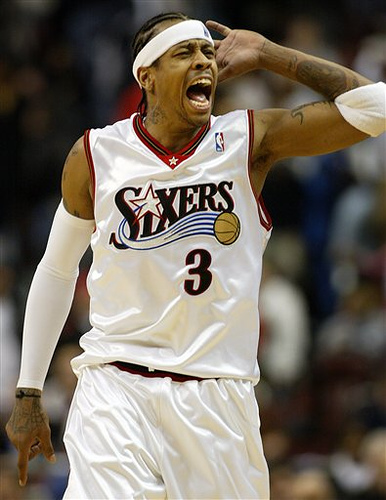A dynamic moment frozen in time captures a Philadelphia 76ers basketball player in the heat of the game. The athlete, donned in a pristine white jersey adorned with dark blue letters spelling "Sixers," is caught mid-yell, his gaze directed to the right. Above the "I" in "Sixers," a white star stands out, a nod to the team's logo. His left hand is extended outward, while his right hand cradles the back of his head, accentuating the intensity of the moment. The front of his jersey features a white and blue swoosh design with a gold basketball emblem, culminating in the prominent number 3 below it.

His right arm is wrapped in a white bandage or cloth that stretches from his wrist to his armpit, a testament to the rigors of the sport. A dark bracelet with yellow accents adorns his right wrist, and tattoos peek out from the back of his hand, with his pointing finger subtly directed downward as his arm rests at his side. The player is clad in white shorts, completing his uniform. In the background, the crowd in the stands is blurred, emphasizing the player as the focal point of this intense scene.